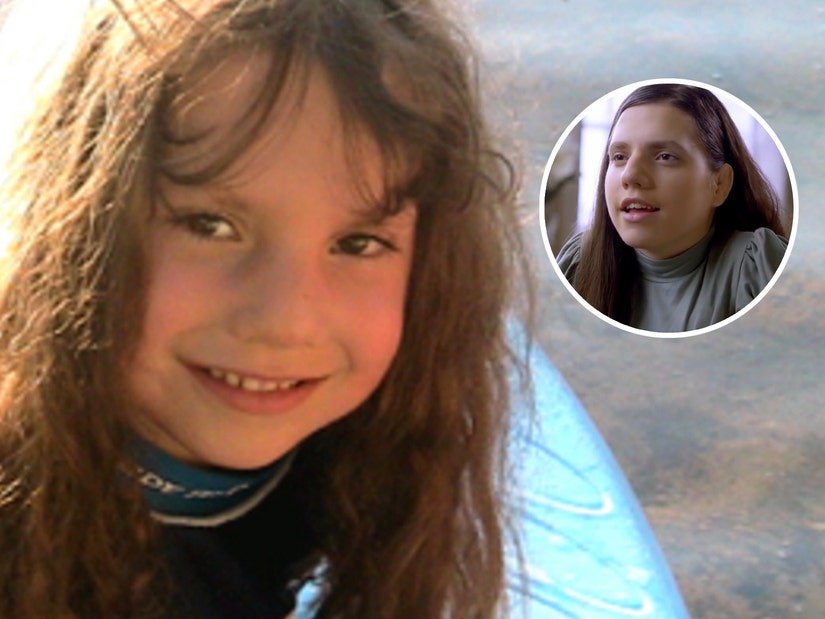In this image, a young girl occupies the left side, showcasing her wide smile with rosy cheeks and brown eyes. Her long, wavy brown hair partially covers a black or blue wetsuit, suggesting she has just had a surf lesson; she appears to be sitting on a light blue surfboard with a backdrop of a marbly surface that reflects water in different shades of blue and gray. In a circular inset on the right, we see an older version of the same girl, now a woman, with long, straighter brown hair parted to the side. She is wearing a green top with slightly puffed sleeves and appears to be mid-speech, looking towards her younger self. This inset likely snipped from a documentary, gives the impression that the woman is reflecting on her childhood. Both images emphasize the continuity of her distinctive eyes, smile, and the settings suggest an aquatic theme, possibly related to an interview or a narrative about her past experiences.